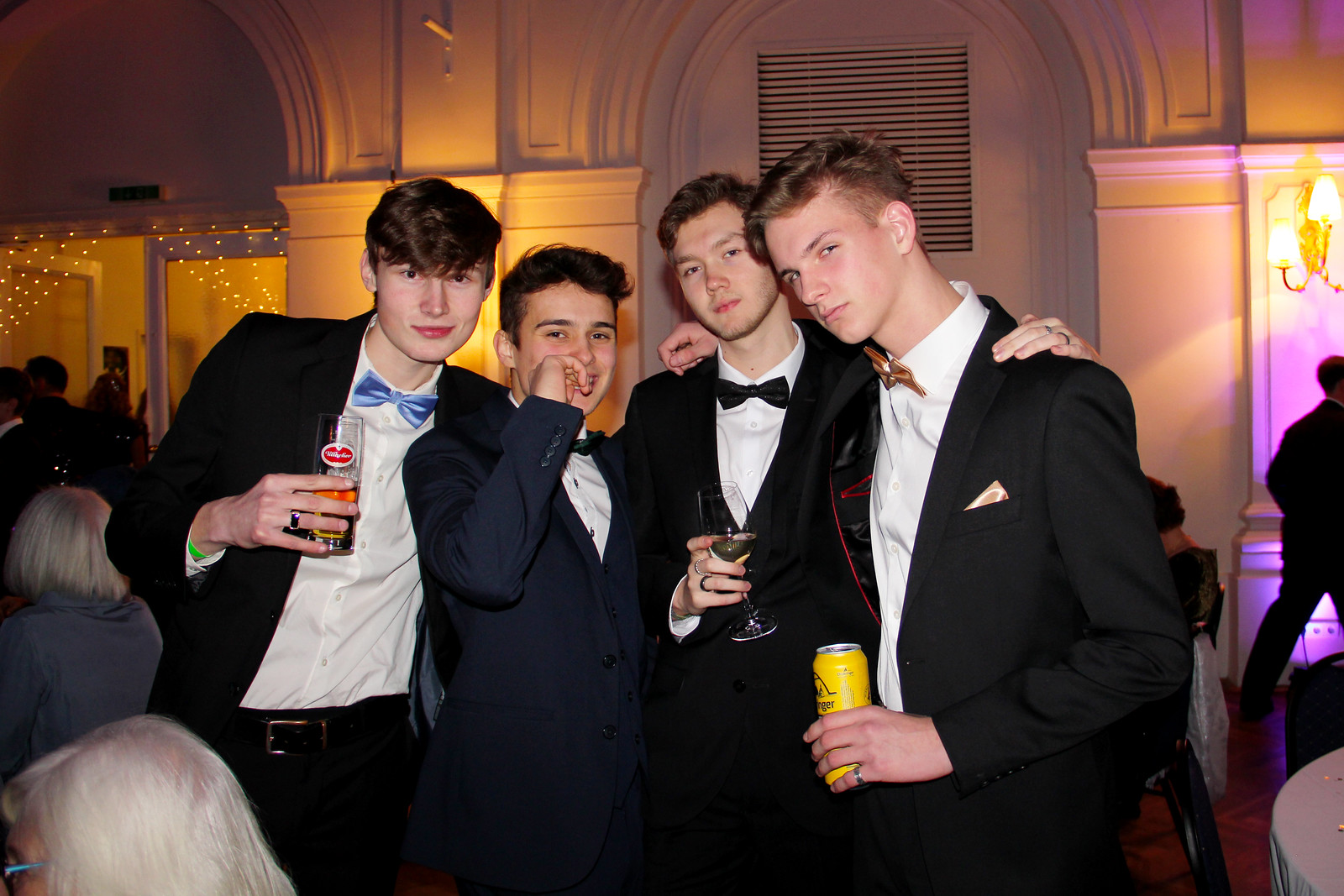This landscape-oriented photograph captures an indoor celebration, likely a prom or wedding, featuring a group of four young men, perhaps teenagers or slightly older, dressed in tuxedos, standing centrally in the image. The setting is an ornate indoor venue with white walls adorned with golden lighting and big arches, alongside string lighting visible near a door on the left.

The four men, each holding a drink, are the focal point. From left to right: 

1. The first man sports a black suit, white shirt, and a distinctive blue bow tie. His reddish-brown hair hangs down to his eyes, and he has his arm around the next person.
2. Next to him, a slightly shorter individual is dressed in a dark blue suit with a white shirt and green bow tie. He has dark brown hair styled in an upward hairdo.
3. The third man wears a black suit, black tie, and white shirt, holding a glass of wine. His dirty blonde hair is combed to one side.
4. The fourth man, on the right, is clad in a black suit with a handkerchief in the pocket, a gold tie, and is holding a large can of what is possibly beer. He has reddish-blonde hair.

In this indoor celebration, the men’s black tuxedos contrast with the white backdrop, while the ornate lighting adds a festive ambiance. Other individuals are visible towards the left and right, contributing to the lively atmosphere.